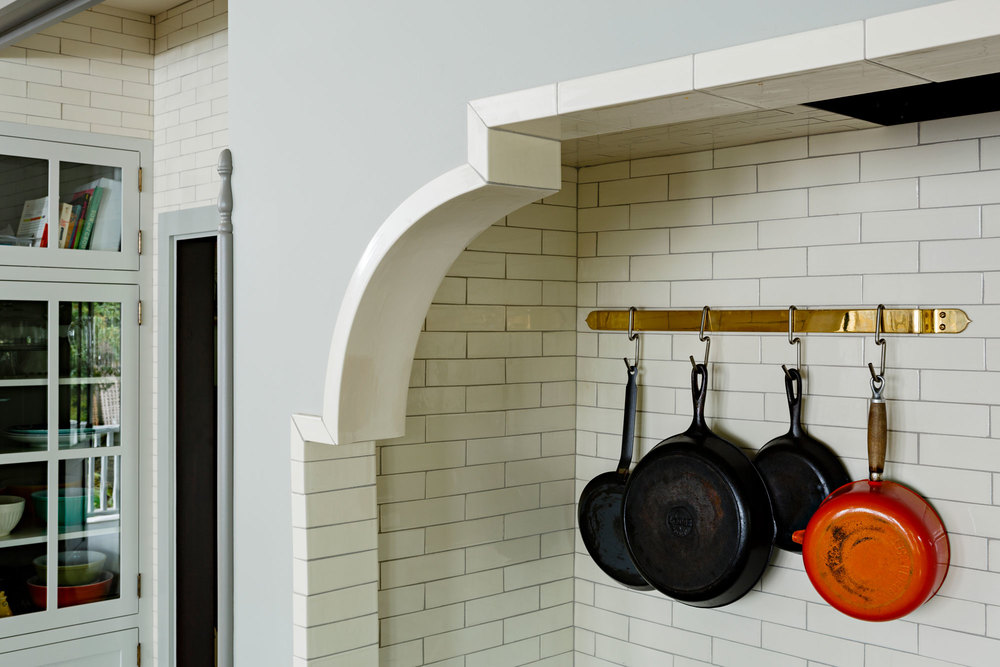The image depicts a cozy kitchen nook featuring a blend of modern and vintage elements. On the left side, there are white wooden cabinets with glass doors, revealing neatly arranged bowls and plates inside. Dominating the central part of the frame, the wall is adorned with white subway tiles laid in a brick pattern. Attached to the tiled wall is a stylish gold-colored rack with four hooks, from which various pots and pans are hanging. The collection includes three cast iron skillets and a distinctive red-orange frying pan with a wooden handle and a silver loop at the end. Surrounding the subway tile, the walls are painted in a soothing grayish blue with matching molding. Additionally, a vent is visible at the lower right side, possibly situated above a stove or a fireplace, adding both function and character to the space. Overall, the image captures the charm and practicality of a well-organized kitchen corner.